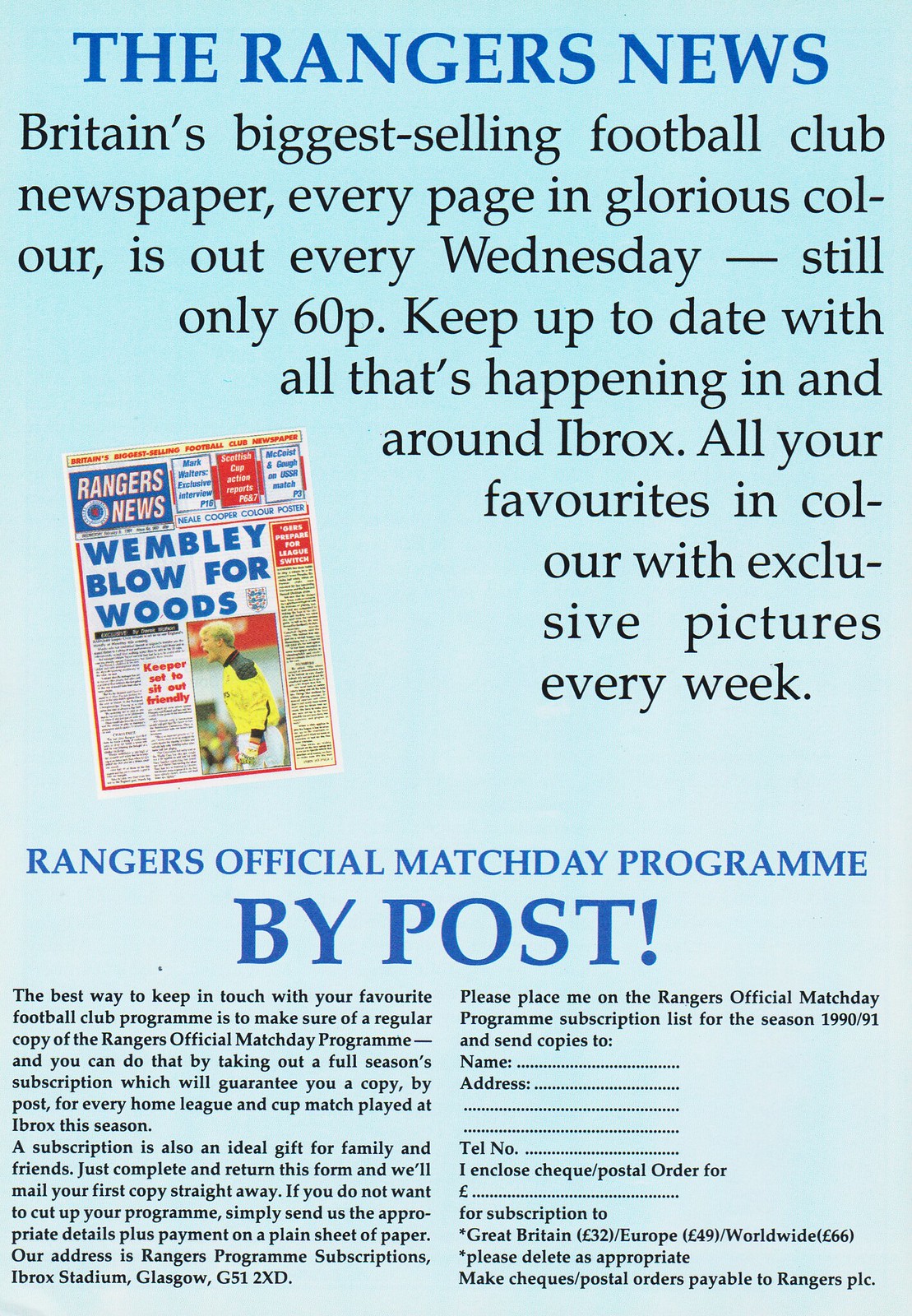The image appears to be a promotional advertisement for "The Rangers News," set against a light blue background. At the very top, in bold dark blue letters, it announces "The Rangers News," followed by "Britain's biggest selling football club newspaper" in black. The promotional text highlights that every page is printed in glorious color and states that the newspaper is out every Wednesday for the price of only 60p. The text encourages readers to keep up-to-date with all that's happening in and around Ibrox, featuring favorite articles and exclusive pictures weekly.

Prominently in the center is a photograph of the newspaper's cover, featuring a headline in large blue lettering, "Wembley blow for Woods." Below this is an image of a blonde goalkeeper in a yellow jersey, white shorts, gloves in hand, screaming, implying intense action or emotion. More headlines detail an exclusive interview with Mark Walters on page 16, match reports on Scottish Cup action on pages 6 and 7, and discussions with McCoist and Gough about a USSR match on page 3. There's also mention of a Neil Cooper color poster and a smaller piece noting girls preparing for a league switch.

In the lower third of the image, another heading in blue states "Rangers Official Match Day Program." Below, it says "by post," emphasizing a subscription service. An accompanying order form invites fans to subscribe to the Rangers official match day program for the 1990-1991 season. Subscribers can guarantee a copy for every home league and cup match played at Ibrox Stadium. The detailed ordering instructions include fields for name, address, and telephone number, and specify payment methods, with subscription prices listed for Great Britain, Europe, and worldwide delivery.

Overall, the image effectively combines visual elements and detailed. promotional text to appeal to fans of The Rangers football club, emphasizing both a weekly newspaper and a seasonal match day program subscription.